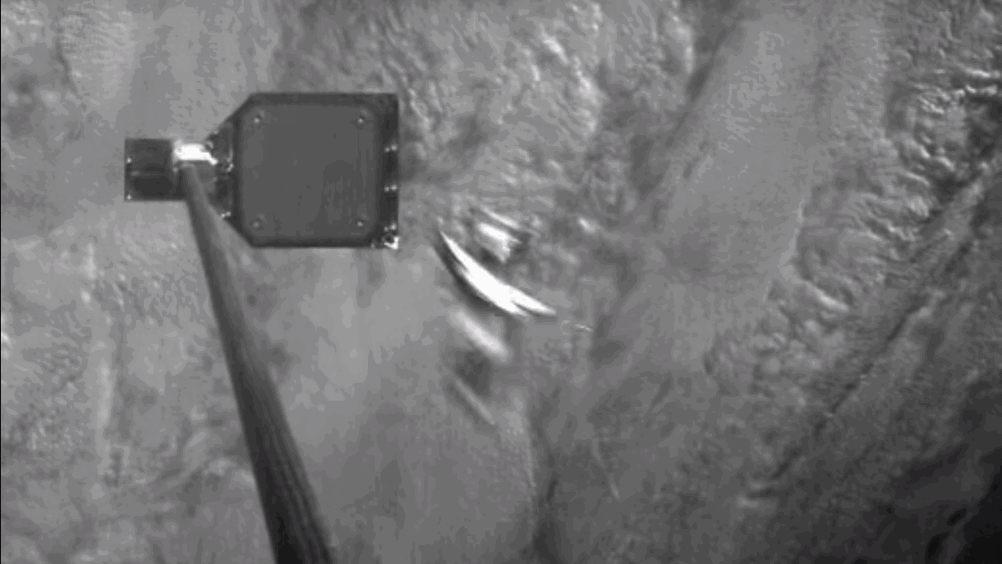This close-up black and white photo presents an intriguing, almost abstract scene. Dominating the foreground is a black metal rod with silver detailing in the middle, emerging from the bottom left of the image. The rod features four screw holes near the base, with a black edging and a small turnable knob also colored black. Just beside the rod, there appears to be an indistinct white shape resembling a bird, adding to the enigmatic nature of the image. The background is difficult to discern; it appears white and possibly cloud-covered, giving a surreal and ethereal feel. The photo is taken from an underside angle, making it look like an aerial or space shot with a cloudy Earth-like surface below. Despite the ambiguity, the sharp details of the rod and its components suggest that the object might be a part of a larger apparatus, possibly a solar panel or a high-tech device. The overall composition creates a mysterious atmosphere, blending mechanical precision with an almost celestial backdrop.